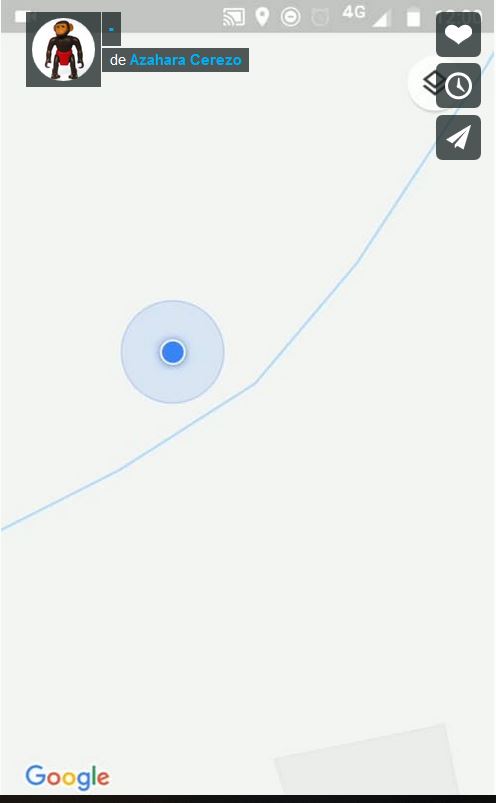This image is a Google Maps screenshot predominantly featuring a blue location dot situated beside a meandering creek that stretches from the middle left to the top right of the frame. The entirety of the image lacks background detail, appearing mostly whited out except for the highlighted stream. In the bottom left corner, the graphic includes the word "Google," with a small black bar immediately below the image. At the top left, there's a square icon displaying an avatar of a monkey at its center, set against a white circular background. Adjacent to this icon, the text "Day Ashara Cerezo" is visible. Overlaying the top of the map image, a series of icons can be seen, including a heart, a clock, and a send icon.